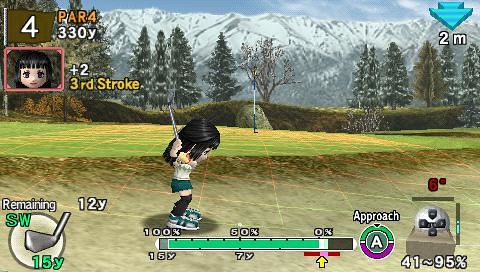This is a color screenshot from the video game "Hot Shots Golf," likely an older-generation game from the late 1990s to early 2000s. The image captures a young girl mid-swing while golfing in a sand trap. She has long black hair and is dressed in a white top with a blue zigzag design, blue shorts, black knee socks, and green and white sneakers. She stands facing to the right, about to strike the ball with a golf club raised over her head. 

The game display shows various details: in the top left corner, it indicates the current hole is a par-4 and the distance is 330 yards. She is on her third stroke and at a plus two score. The bottom left corner features a circle containing a sand wedge icon and notes the remaining distance as 12 yards to the hole, with her current swing aimed at 15 yards. There's also a power meter showing her swing strength and direction, with the top right corner displaying the wind speed blowing at two miles per hour against her. 

The background features a picturesque golfing scene with a flagpole marking the hole on a green area, fir trees dusted with snow, a snow-covered mountain range, and a hint of blue sky above. The sand trap she's in has distinct lines marking the sand, adding realism to the game environment.